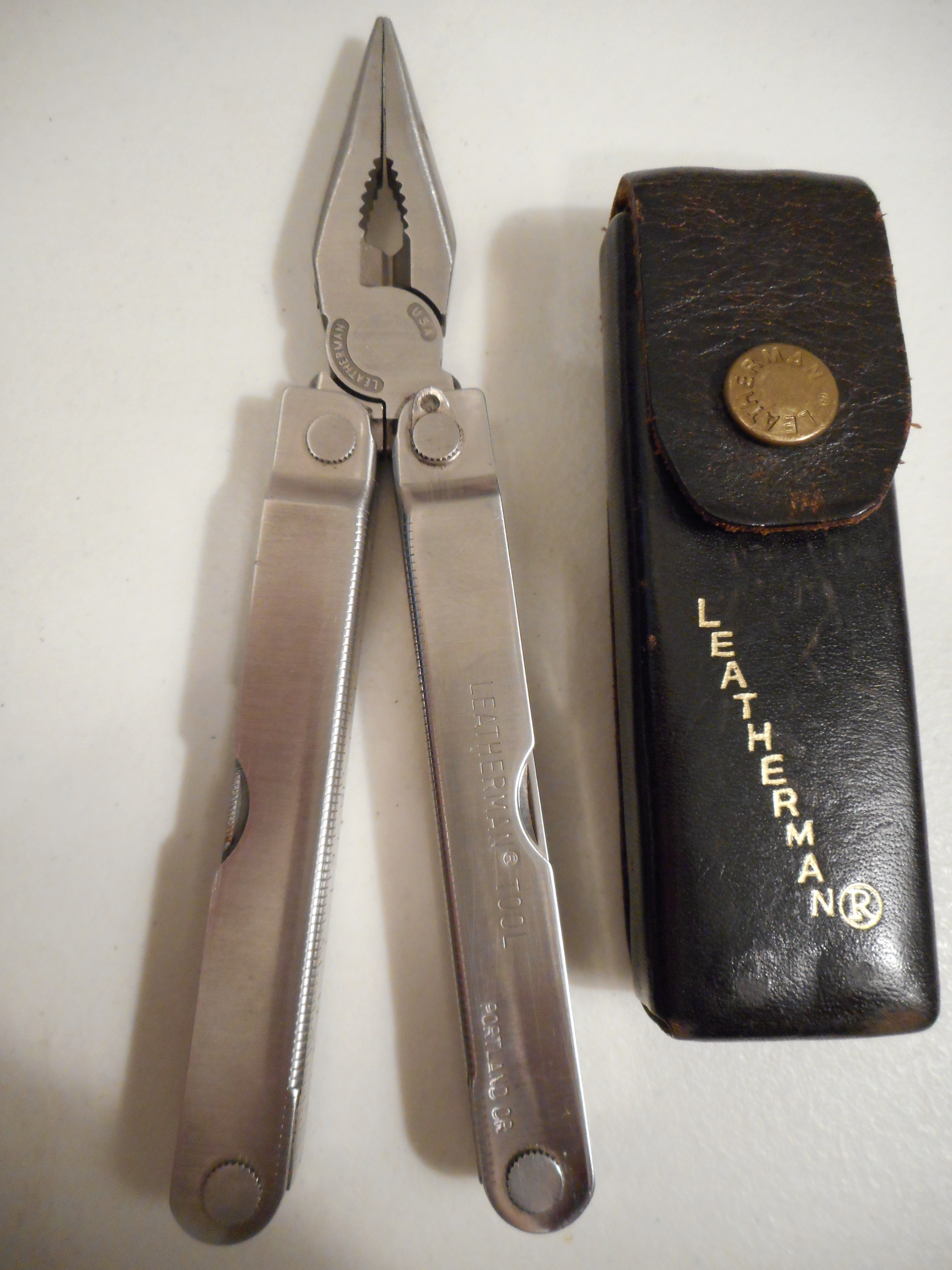This close-up photograph features an older pair of stainless steel Leatherman pliers set against a white backdrop. The pliers, which are currently closed, display intricate details like visible rivets and fine etchings. The etching on the handles reads "Portland, Oregon" alongside the brand name, "Leatherman." The tool's design includes serrated jaws and suggests multi-functionality with sections in the handles where additional tools like knives or nail files could be housed. To the right of the pliers lies a closed, black leather sheath with a vertical gold Leatherman logo and a button clasp embossed with the brand name, reminiscent of a button on a Levi’s jacket. The sheath is rectangular and suggests that it might fit the pliers if they are foldable.